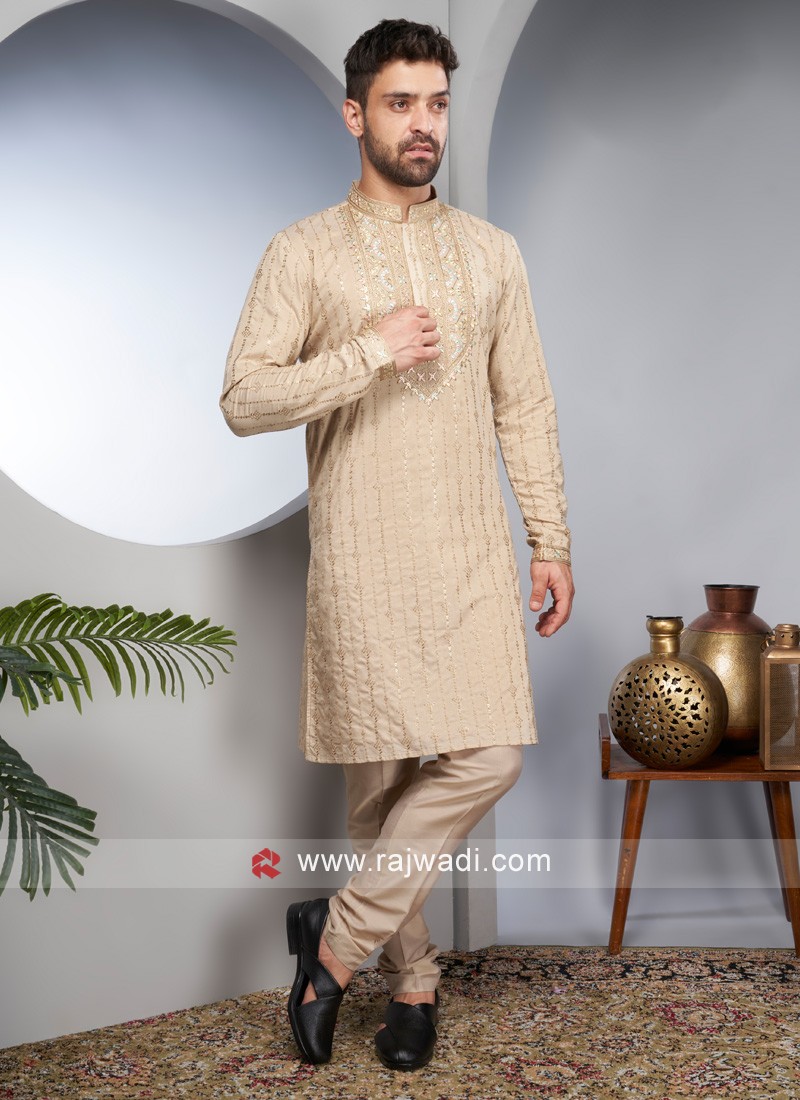In this detailed image, a man, possibly an Indian model with short, dark hair, and a neatly trimmed beard and goatee, stands dressed in a traditional, long, tan-colored kurta that reaches down to his knees. He pairs the kurta, embellished with subtle jewels, with light cream-colored pants and black dress shoes, without socks. The man is standing in a predominantly gray room, featuring decorative gray circular cutouts behind him. To his right, there's a small brown wooden table adorned with golden vases and various decorative containers. The room is further accented with a floral or abstract patterned rug enhancing the elegant décor. Additionally, a plant can be spotted on the left side of the image. At the bottom of the photo, the website www.rajwadi.com is visible, possibly a branding element, along with a red logo resembling a "Q."